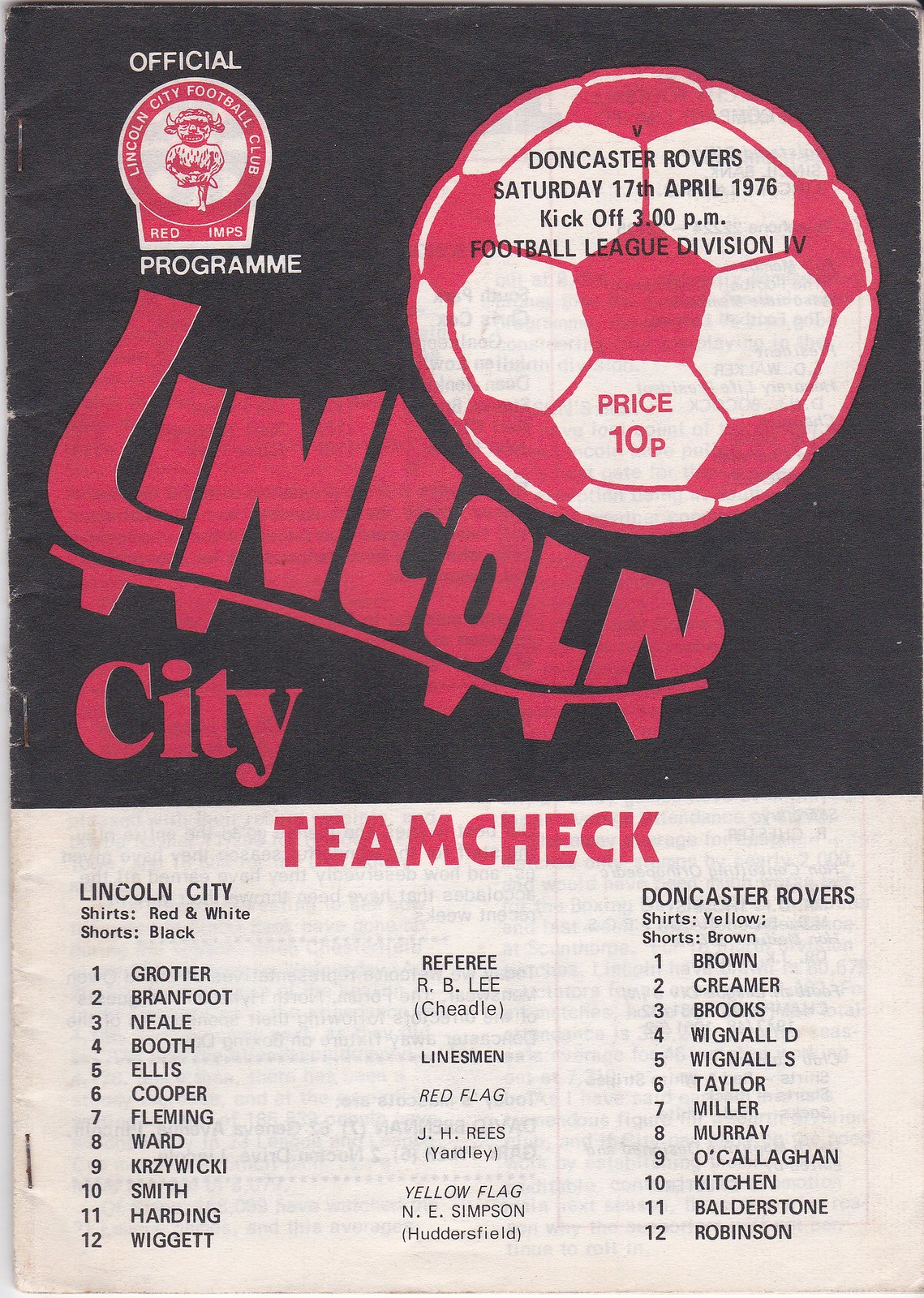The image depicts an official program for a football match between Lincoln City Football Club and Doncaster Rovers, dated Saturday, 17th April 1976, with a kickoff time of 3 p.m. The program's top half features a black, red, and white color scheme, showcasing the word "Lincoln" stylized as a football cleat. Adjacent to this, in the top right corner, is a red and white soccer ball with inscriptions detailing the opposing team, Doncaster Rovers, and match particulars including the date, time, division (Football League Division IV), and price (10p). Below this, in bold red letters, is "Team Check," beneath which the rosters for each team are listed: Lincoln City players on the left wearing red and white shirts with black shorts, and Doncaster Rovers players on the right in yellow shirts with brown shorts. The center of this section includes details of the referee and linesmen. The program's overall design has an upper section in a black and red palette, while the lower section is predominantly white with prominent red and black text.